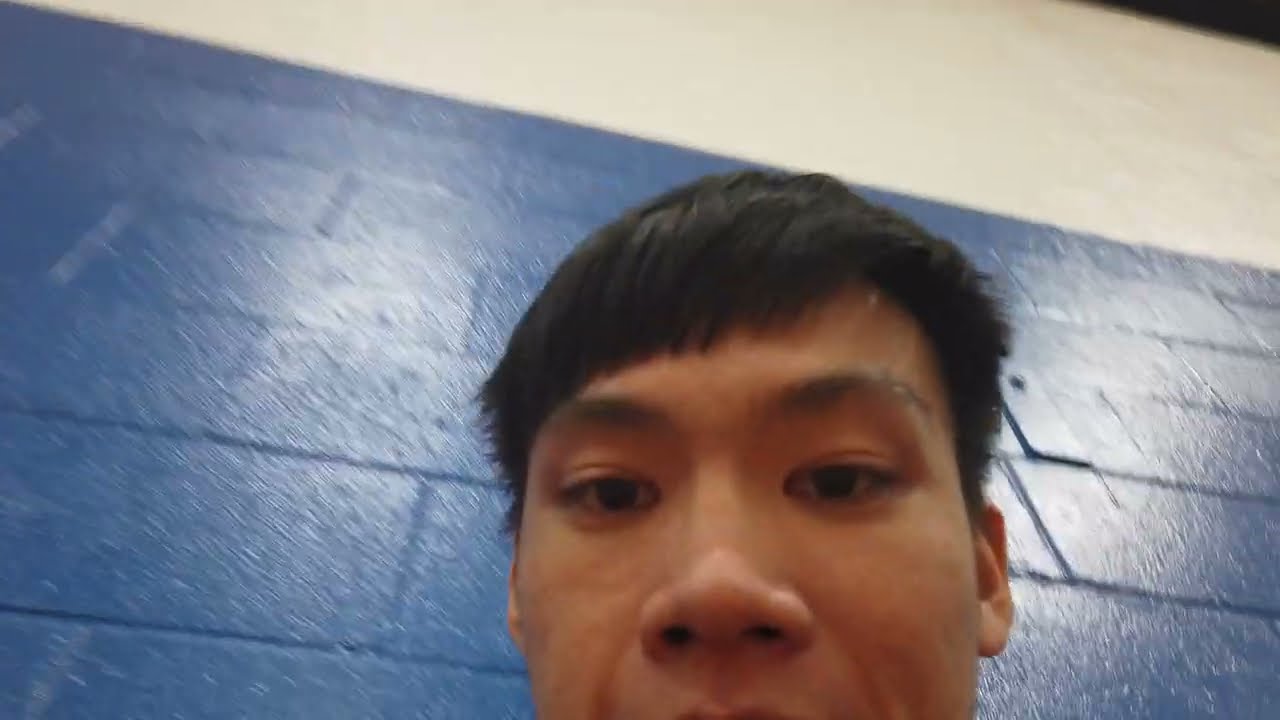In the image, a young man with tan skin and short black hair is taking a selfie with a camera that is angled slightly upwards, resulting in only the top part of his face being visible from his nose upwards. He is looking down towards the camera, and his hair is brushed to the left. Behind him is a brick wall that adds a contrasting backdrop with its distinct halves: the lower part is painted blue and the top half is a light beige color. The framing of the picture includes bright reflections from ceiling lights on the blue section of the wall, creating a dynamic and tilted visual effect. There's also a noticeable small black triangle in the upper right-hand corner of the wall, contributing to the geometric composition of the background.